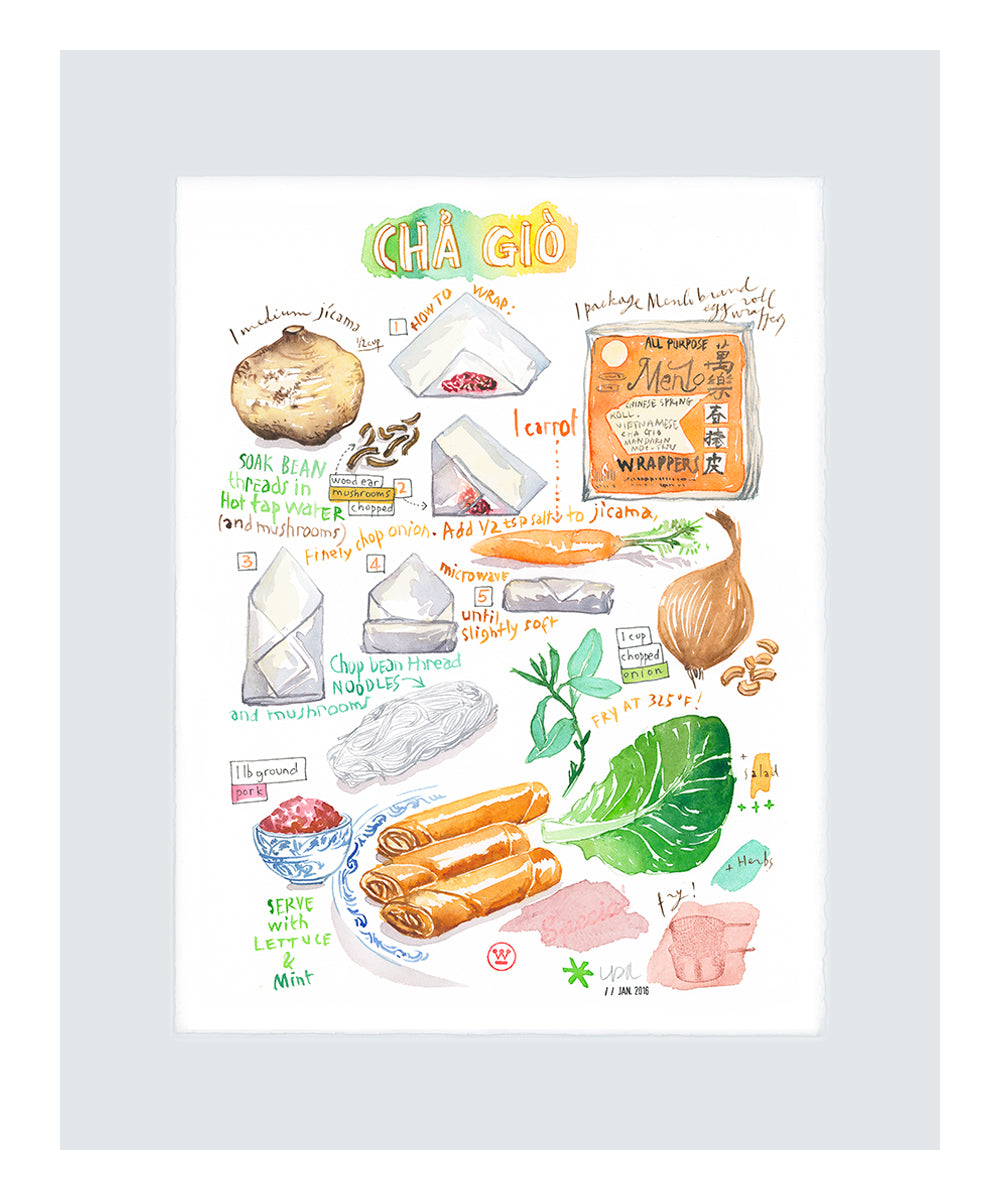The image is a detailed watercolor poster, bordered by a light gray mat, and showcases how to wrap a spring roll. At the top, "Chai Gio" is written with "Chai" on a green background and "Gio" on a yellow background, highlighted by a rainbow watercolor backdrop. Below this, the poster offers step-by-step instructions on wrapping a spring roll, with visuals and text to guide the process. Key ingredients and food items illustrated include vegetables like carrots, bok choy, jicama, and onions, along with instructions to soak bean threads in hot tap water and chop onion, pork, and mushrooms. It also shows finished spring rolls, wrappers, and specific cooking tips such as frying at 325 degrees. The colorful, artistic collage combines various ingredients and steps, making it both visually appealing and informative.